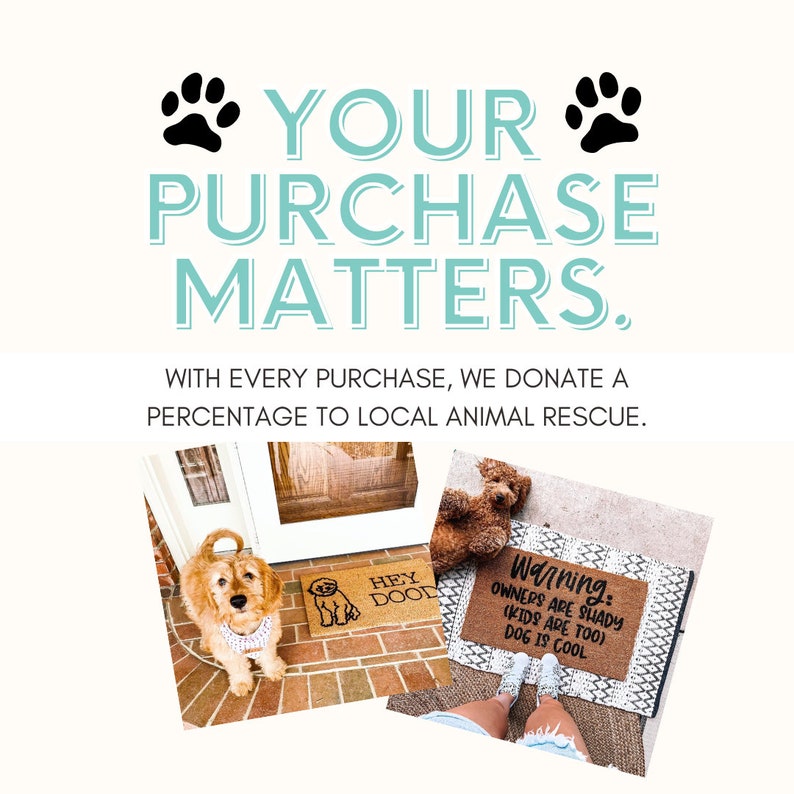**Descriptive Caption:**

The advertisement presents a warm, inviting layout with a pale pinkish background. Positioned at the top of the ad, the phrase "Your Purchase Matters" is prominently displayed in teal, flanked by black paw prints on either side. Below this central message, another line of text in black reads, "With every purchase, we donate a percentage to local animal rescue."

Two images are featured prominently in the ad:

1. The first image captures a small, scruffy-looking blonde dog with black eyes and a black nose, standing proudly on a brick entryway outside a front door. The dog is adorned with a white collar or possibly a harness. The background includes an orange wood front door, a white storm door, and a welcoming tan doormat with the phrase "Hey Doodle" in black, accompanied by a simple black outline of a dog.

2. The second image shows a person's legs clad in ragged denim shorts and white shoes, standing on a black and white Chevron patterned mat. The mat has a tan section that humorously states, "Warning, owners are shady, kids are too, dog is cool," in black text. At the bottom of the image, a caramel-colored stuffed animal dog with black eyes and a black nose is visible, resting on a gray carpet.

These images collectively highlight a cozy, pet-friendly home environment with a touch of humor and a focus on supporting local animal rescues through consumer purchases.